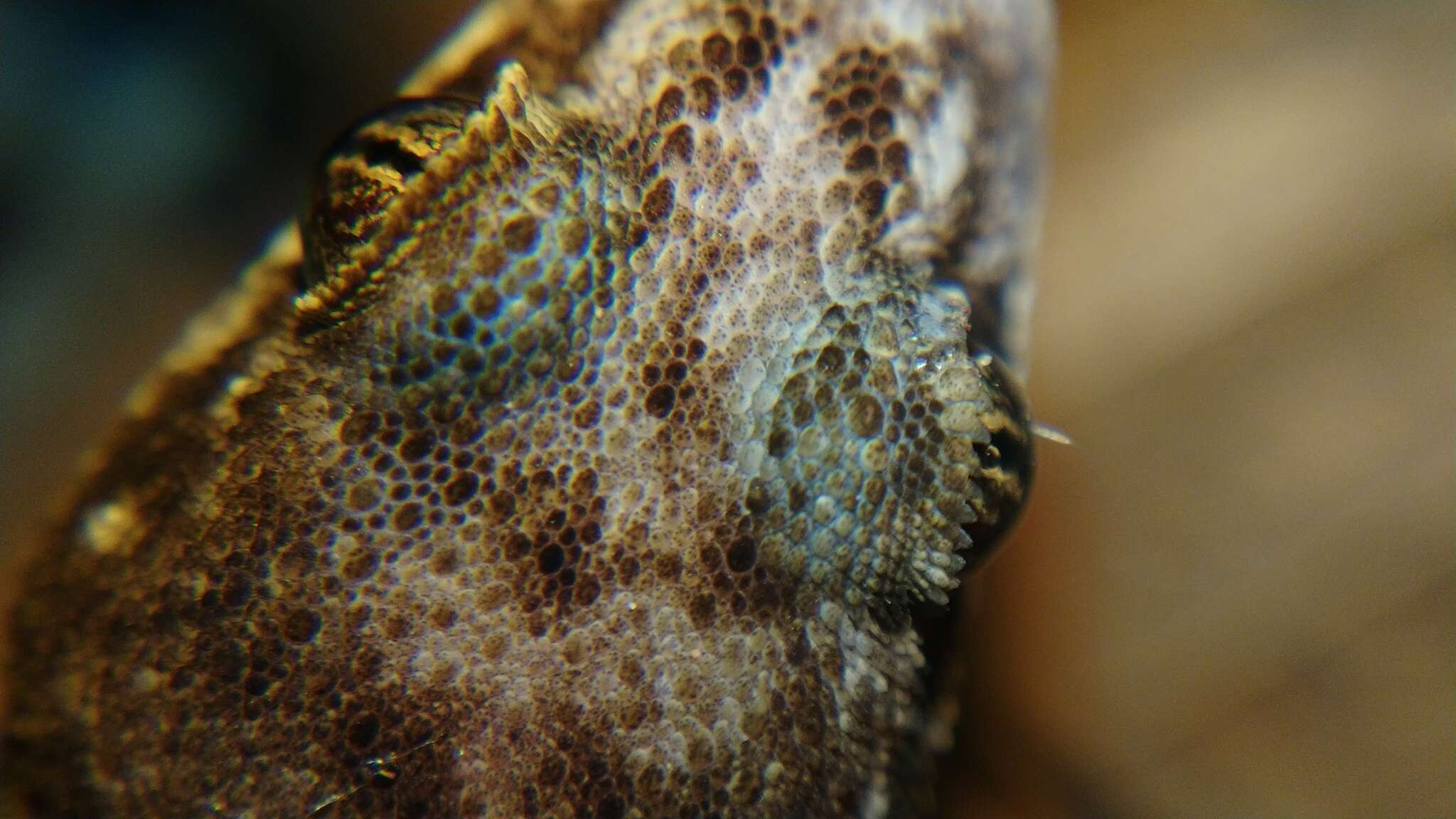The photograph captures a close-up of a reptilian head, likely a small lizard, viewed directly from above. The head is predominantly covered in beige, brown, and cream-colored scales with hints of grayish-green and golden tones. The animal's bulging eyes, which are vivid gold with narrow black pupils, are prominent features positioned on either side of its narrow head. While the background is blurred and indistinct, potentially natural or fabricated, it does not detract from the detailed texture and coloration of the reptile’s scales and striking eyes. This meticulous composition centers on the reptile’s eye area, emphasizing its vibrant appearance and suggesting the creature’s alertness and life.